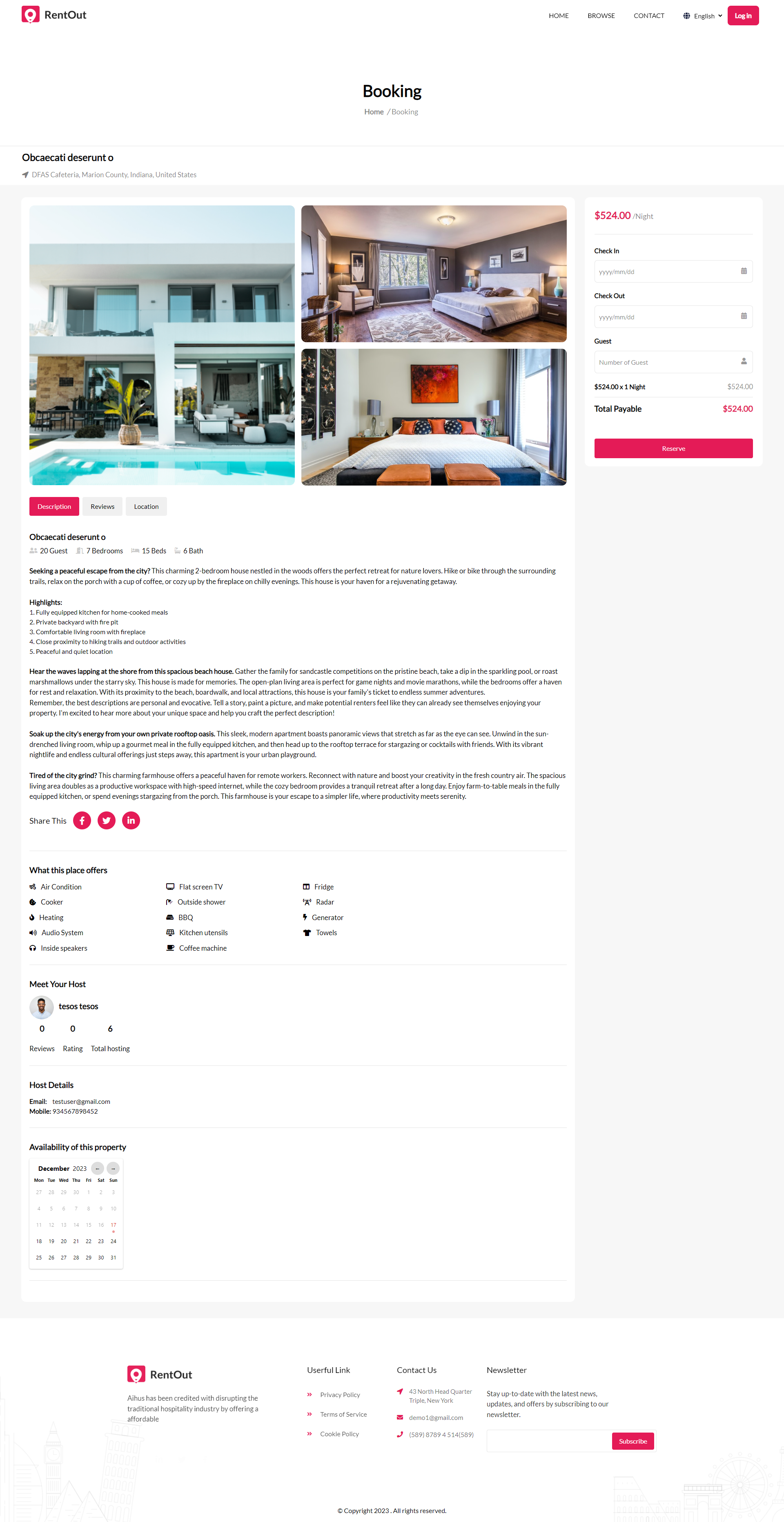The image depicts a booking page, which closely resembles an Airbnb listing. At the top of the page, there is a red logo featuring an indiscernible icon within a circle. Beside the logo, in black font, the text likely reads "Rent Out," flanked on the right side by menu options including "Home," an unreadable item, possibly "Contact," and a "Login" option. Adjacent to these is a prominent red button with white text.

The title "Booking" is displayed prominently in bold black font, with some additional information below it in gray, though it cannot be read clearly. Further down the page, the listing name, also in bold black font, comprises two words.

The listing presents three images of the property. The first image shows the entire house from the backyard, revealing a two-story building with a swimming pool and a back patio. The second image, positioned to the right, appears to be the master bedroom. The third image, located just below, showcases an additional bedroom.